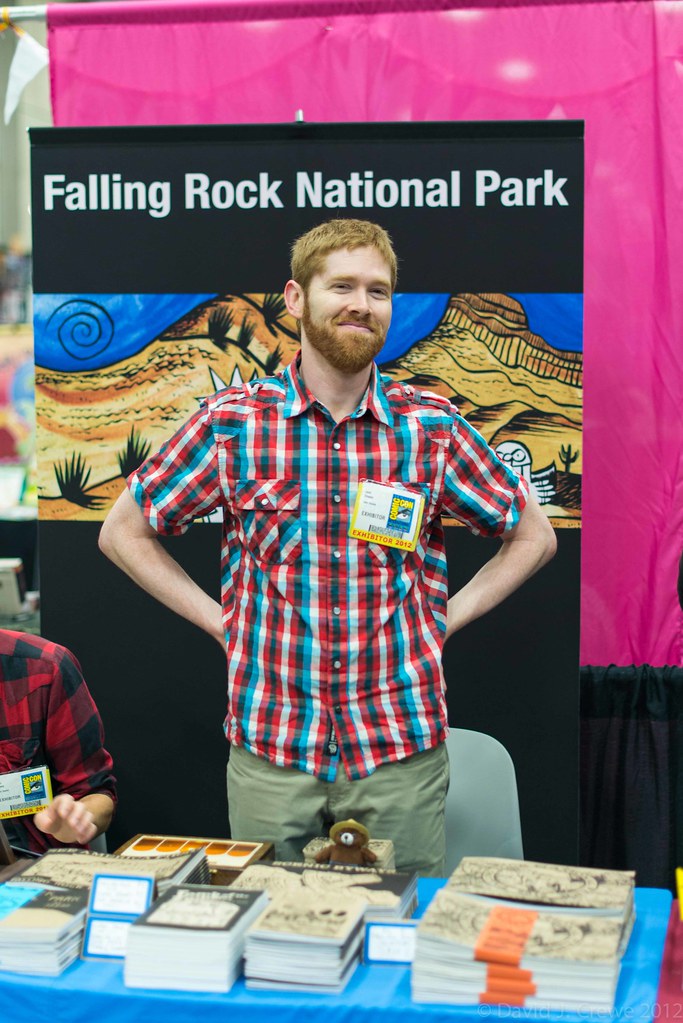In this photograph, a smiling young man with red hair and a matching beard stands confidently with his hands on his hips, in front of a booth brimming with neatly organized books and pamphlets. He wears a blue, white, and red checkered short-sleeve shirt, which gives off a cowboy vibe, and has a name tag affixed to the left chest pocket. His pants are green khakis, complementing his casual, approachable appearance. The booth is set against a backdrop featuring a sign that reads "Falling Rock National Park" in white text on a black background, with an abstract painting below depicting arid, orange mountains dotted with cacti and other desert flora under a blue sky. There’s a prominent stuffed Smokey the Bear toy placed atop one of the piles of books on the table. A partially seen man in a black and red checkered shirt sits to his left, his face out of frame. The scene is completed by a pink curtain to the right, adding a touch of color to the background.